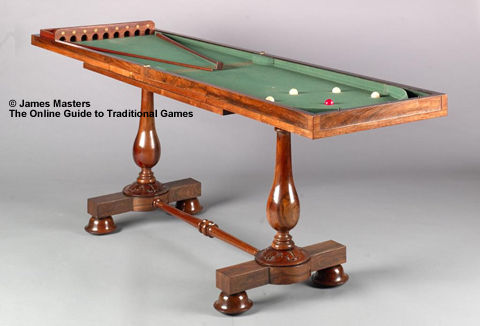This photograph captures a vintage snooker-like table with a green felt top and medium-colored, lacquered wooden sides. The table isn't full-sized; rather, it's more compact, suggesting portability. It features four teardrop-shaped wooden legs with circular bases, all connected by a central wooden pole. The table’s upper surface showcases four small white balls and one red ball arranged in a semi-arc. At one end of the table, there are eight arching black holes meant for gameplay. A distinctive V-shaped wooden piece rests on the felt. The text “Copyright James Masters, The Online Guide to Traditional Games” is inscribed on the side, further emphasizing its connection to traditional gaming.